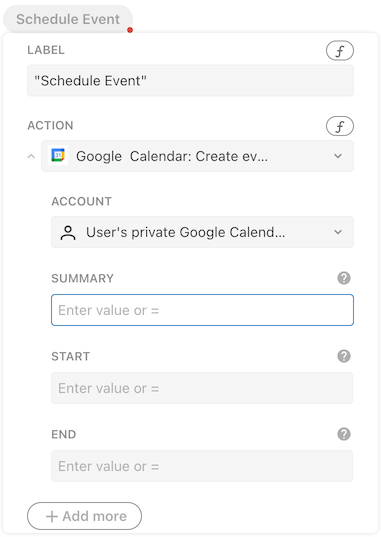This screenshot displays a detailed view of a scheduled event creation interface on a mobile device using Google Calendar. The interface prominently labels the event entry as "Schedule event." The action assigned to this event is "Google Calendar create event," indicating that this task is set to add a new event to a Google Calendar.

The account associated with this action is the user’s private Google Calendar, suggesting that the event will be added to their personal calendar. The interface includes various input fields:

1. **Summary:** This field prompts the user to "Enter value or equal," indicating that they need to provide a title or description for the event.
2. **Start:** Similar to the Summary field, this field requires the user to "Enter value or equal," which likely refers to the start time and date of the event.
3. **End:** This field also asks the user to "Enter value or equal," for specifying the event's end time and date.

There is an "Add more" button, suggesting the option to include additional details or parameters for the event. Above the input bars are function buttons that could offer additional features or settings for the event.

To the right of the "Schedule event" label is an additional function button. This button probably provides extra options or settings related to the event entry.

The action configuration, labeled as "Google Calendar create event," includes a drop-down button, which implies that the user can tweak the event creation settings or change the action entirely to suit their preferences.

Additionally, the interface allows the user to select the account under which the event will be created, which is useful for those managing multiple accounts. This feature enhances the user's ability to stay organized and receive appropriate notifications.

Overall, this screenshot represents a robust event scheduling interface within Google Calendar, equipped with various customizable options to cater to the user's planning needs.